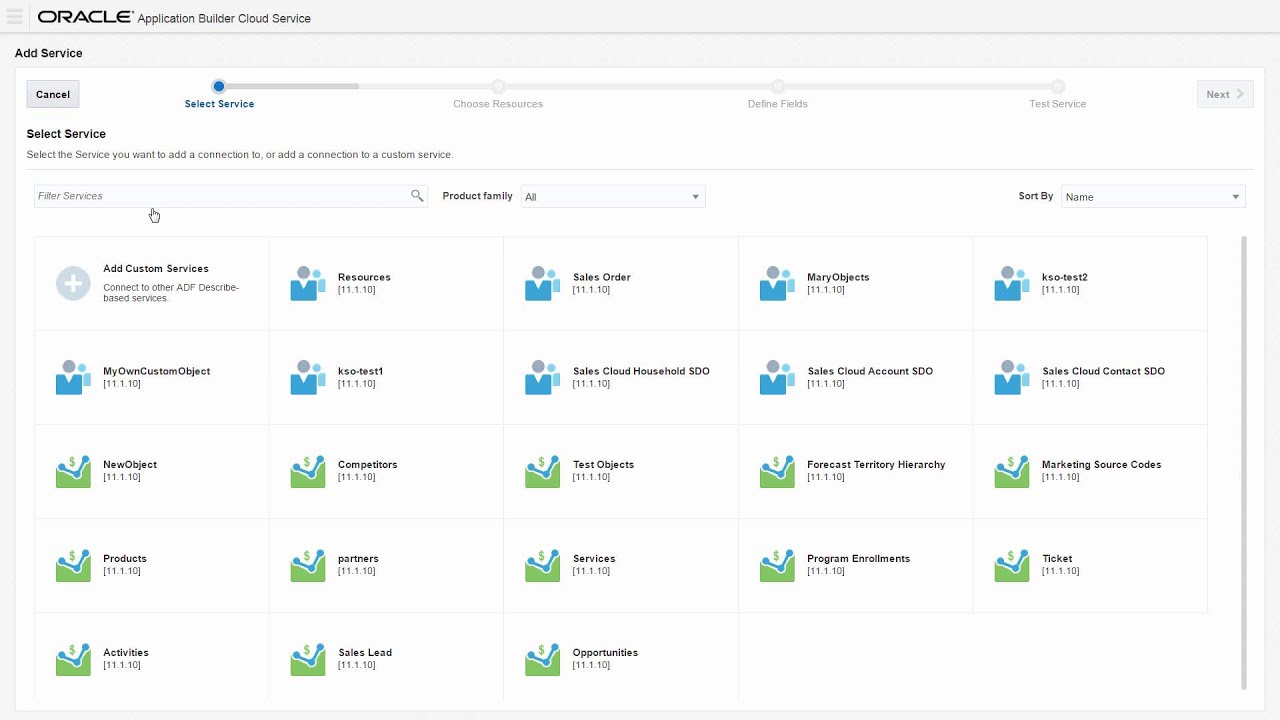The image depicts the Oracle Application Builder Cloud Service interface, specifically showcasing the selection process for adding various services. The interface is divided into several sections. 

At the top-left corner, the Oracle logo is prominently displayed. Below it, a header reads "Add a Service", indicating the current step in a multi-step process, visually represented by a progress bar featuring a series of dots. The first dot, titled "Select Service", is filled in with blue, showing the user's current step, while the subsequent dots, labeled "Choose Resources", "Define Fields", and "Test Service", remain unfilled, signifying upcoming steps. Near the top right corner, a right-pointing arrow labeled "Next" suggests moving forward in the process, while a "Cancel" option to the left of the progress bar allows the user to exit this process.

Below the header, instructions prompt the user to "Select the service you want to add a connection to or add a connection to a custom service". A search bar is provided to filter available services, accompanied by controls to narrow results by "Product Family: All" and sort them "Sort by Name". Additionally, a plus ("+") button allows the user to "Add Custom Services" and to "Connect to Other ADF Described Base Services."

The main section of the interface presents a list of services available for selection. Each service features an icon, with various icon designs, predominantly in blue and green color schemes. Icons include representations of people and dollar signs. The list of services includes "Resources", "Sales Orders", "Merry Objects", "My Own Custom Object", "KSO Test 1", "Services", "Partners", "New Objects", "Products", "Sales Lead", and "Opportunities", among others. This visual organization helps users quickly identify and select the specific service they need for their application.